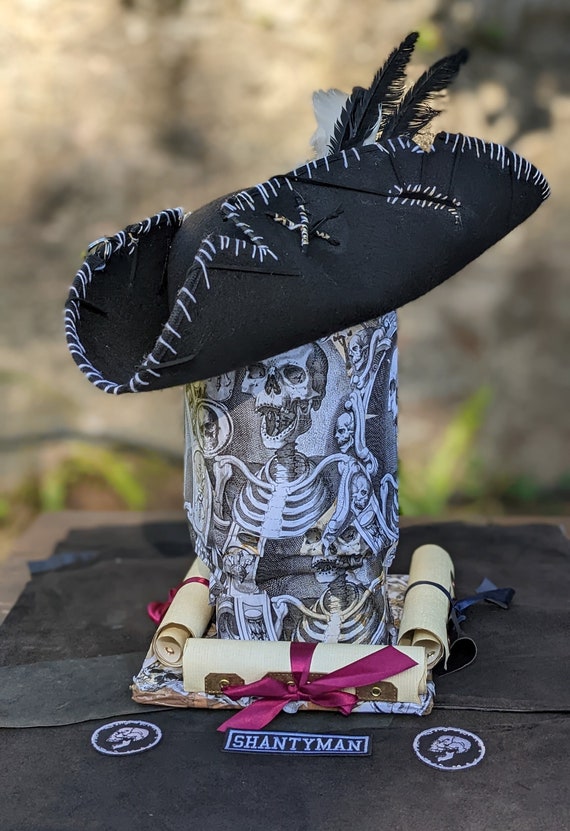This is a vertically oriented, realistic photograph taken outdoors, evident from the brown and green grasses and dirt in the background, bathed in sunlight. In the foreground, a wooden table is set with a black cloth. Centered on the table is a display featuring an intricate piece of art. The centerpiece is a black and white cylinder adorned with images of skeletons. Crowning this cylinder is a black pirate hat from the 1700s or 1800s, decorated with black and white feathers and white stitching. Below the cylinder is a white base holding three cream-colored scrolls with metal ends: one scroll tied with a black ribbon and two tied with maroon ribbons. A sign with a black background and white trim, bearing the text "Shanty Man," is also part of the display. Additionally, there are two circular patches—one on the left and one on the right—both featuring a black background with a white skull motif. The cohesive arrangement suggests a pirate-themed exhibit or art piece.